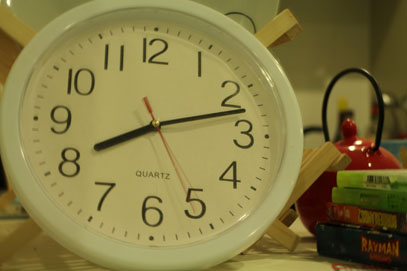This image depicts a neatly organized table or countertop scene. Centrally, there is a clock with a white rim. The clock face is traditional, featuring black hour and minute hands, a red second hand, and standard numbering with 12 at the top, 6 at the bottom, 1 through 5 on the right side, and 7 through 11 on the left. The clock displays the time as approximately 8:12, with the second hand positioned directly on the 5 mark.

To the left of the clock, there is a stack of four items, likely books or board games. The stack includes two green items at the top, followed by a red one, and a bluish-black one on the bottom, which bears the name "Raymond" on its spine.

In the background, there is a red tea kettle resembling a teapot. Behind it, wooden slats suggest the presence of a drying rack typically used for air-drying dishes. The overall setting appears cozy and organized, combining elements of functionality and decor.